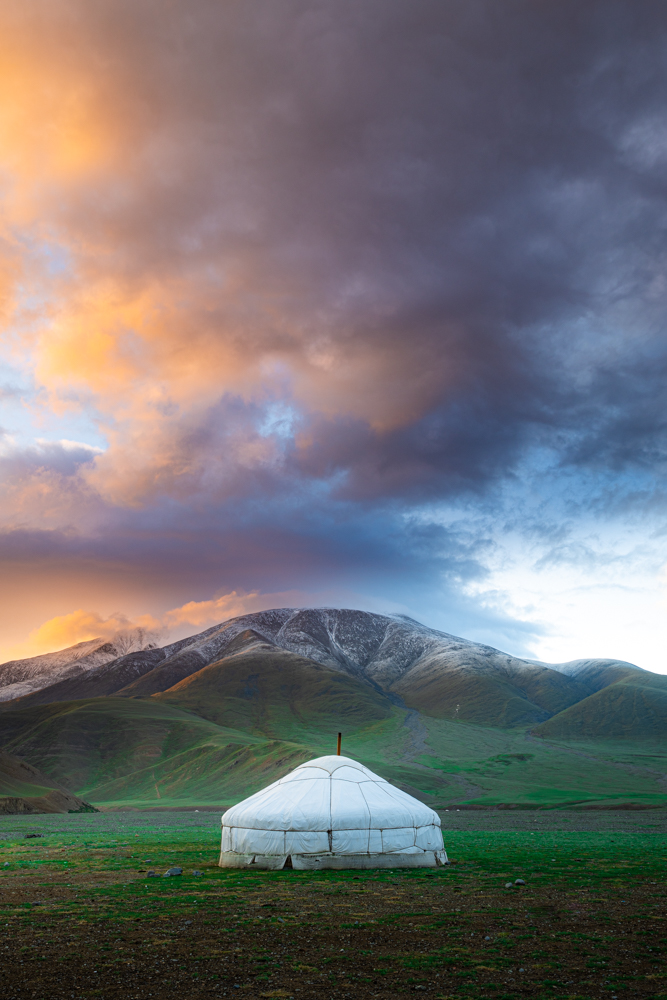The photograph captures a serene outdoor landscape with a prominent white tent, resembling a yurt, positioned at the center of the image. The tent, characterized by its cylindrical base and conical roof, is set on a vast, flat expanse that alternates between patches of green grass and brown soil. Surrounding the tent is a sprawling, open field that conveys a sense of tranquility and spaciousness. In the background, a range of rolling mountains forms a picturesque backdrop. The mountains feature green and brown hues at their base, gradually transitioning to snow-capped peaks. The sky above is a dramatic display of colors with dark, heavy clouds interspersed with bits of bright blue and tinges of orange and gray. The overall clarity of the image is sharp and bright, accentuated by the natural daylight that illuminates the scene, highlighting the vibrant details of the landscape.